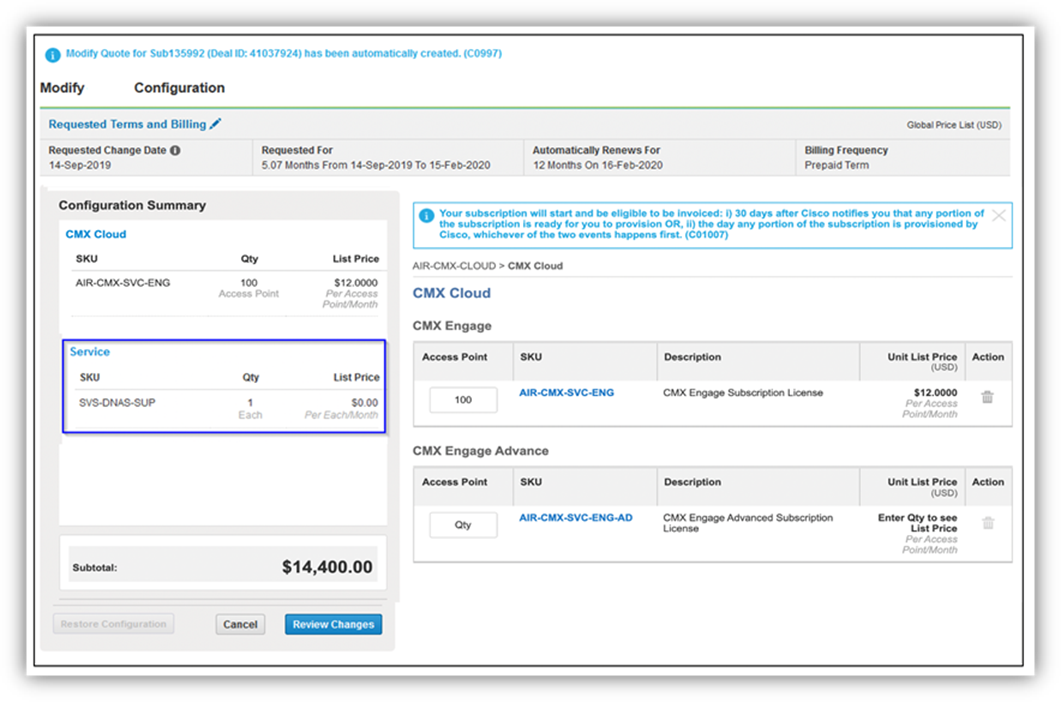In the upper left corner, the text "Modify Quote for Sub 135992, Deal ID 41037924 has been automatically created (CO997)" is displayed in bright blue. Below that, "Modify Configure" is indicated. A green line follows, leading to the section titled "Terms." Under "Requested Terms and Billing," it shows a change date of 14 September 2019. The request is for a duration of 5.07 months from 14 September 2019 to 15 September 2020, with an automatic renewal for 12 months on 15 February 2020.

An information summary is provided with details:
- CMX Cloud SKU: AIR-CMX-SVC-ENG
- Quantity: 100 access points
- List Price: $12,000 per access point per month

Additionally, for the services:
- SKU: SVSDNAS-SUP
- Quantity: 1H
- List Price: $0.00 per month

The subtotal amounts to $14,400. At the bottom, options to "Review Changes" and "Cancel" are available.